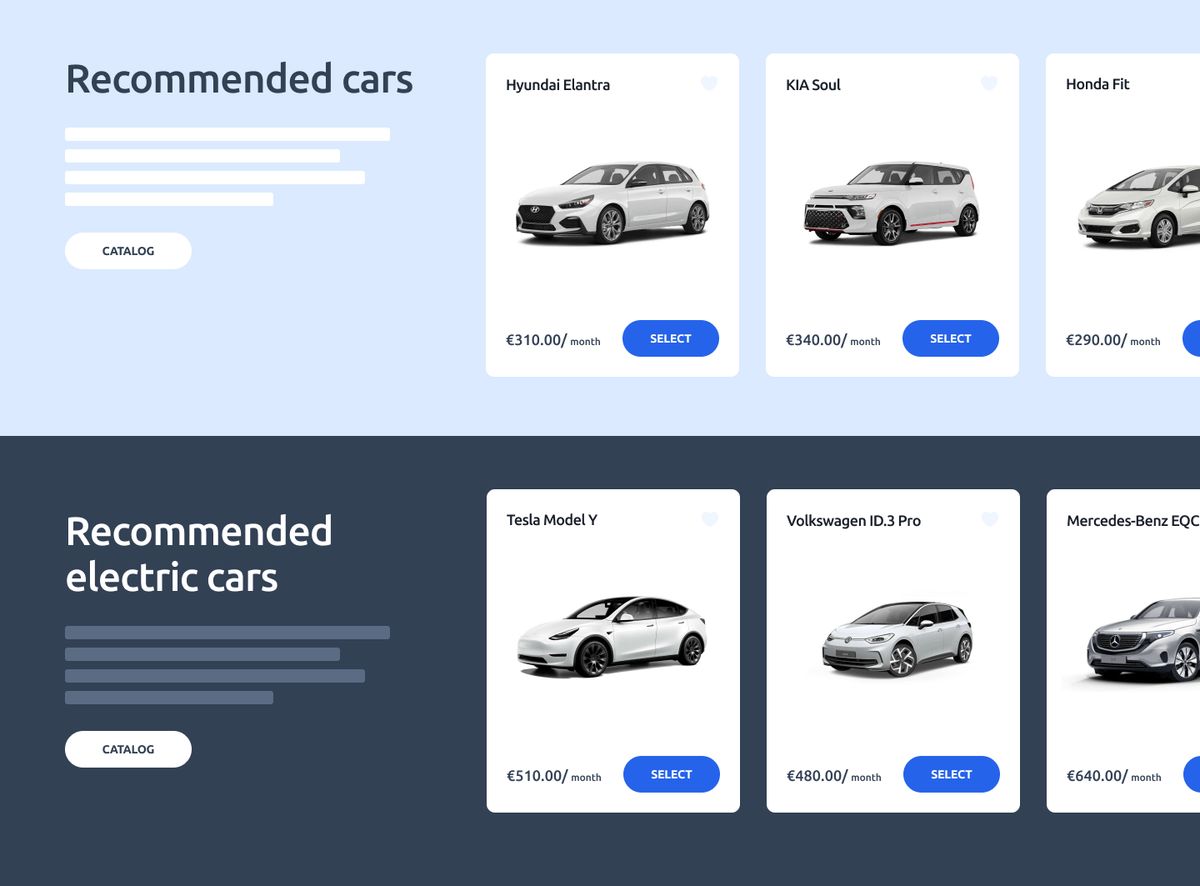In this image, the upper left-hand corner displays the heading "Recommended Cars". Below this heading are four lines where placeholder text in the form of white rectangles is situated. Beneath these rectangles, there is a button labeled "Catalog". On the right side of the image, three cars are displayed in sequence with their names and blue "Select" buttons in the bottom right corner of each. The first car listed is a Hyundai Elantra, followed by a Kia Soul, and finally a Honda Fit.

The bottom section of the image is labeled "Recommended Electric Cars". Similar to the upper section, this part also contains white rectangle placeholders beneath the text and another "Catalog" button on the left side. This section presents three electric cars: a Tesla Model Y, a Volkswagen ID.3 Pro, and a Mercedes-Benz EQC, each accompanied by a blue "Select" button in the bottom right corner.